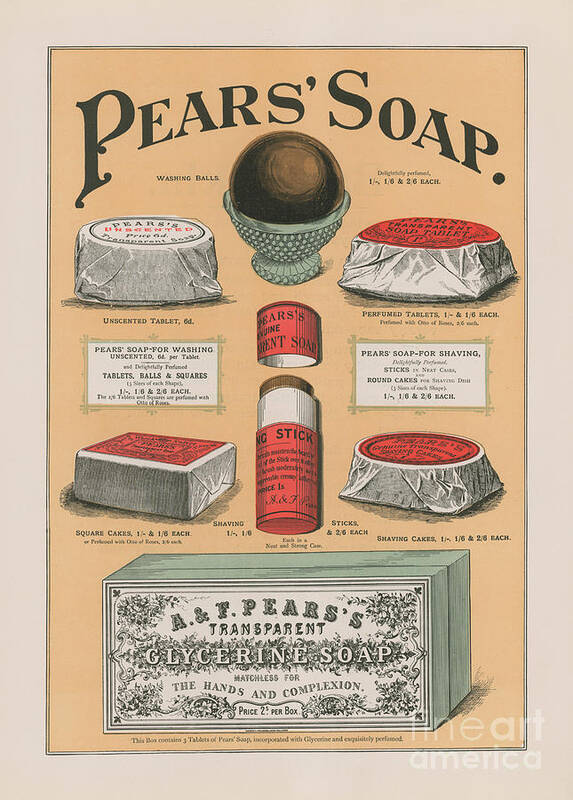This vintage advertisement, which could be from a magazine or a poster, promotes Pears' Soap using a detailed and ornate design. The image is set against a light peach-colored background, framed by a delicate double black line and a beige border that highlights the central content. At the top, there's large, arched serif text reading "Pears Soap." The advertisement showcases a variety of soap types, all packaged with the Pears branding. These include two disks of soap positioned to the right and left, labeled as unscented tablets and perfumed tablets, as well as spherical washing balls.

As the eye moves downward, the layout features additional products such as shaving sticks and square cakes of soap, each illustrated with their respective packaging except for the washing balls, which are shown bare in a green dish. Towards the bottom, a prominent box of A&F Pears' Transparent Glycerin Soap is displayed with an intricate black and white filigree design. The box is marked with the tagline "Matchless for the Hands and Complexion." The price listed is $2.50 per box. This elaborate and richly detailed advertisement, with its turn-of-the-century aesthetic, effectively captures the timeless elegance and quality associated with Pears Soap.